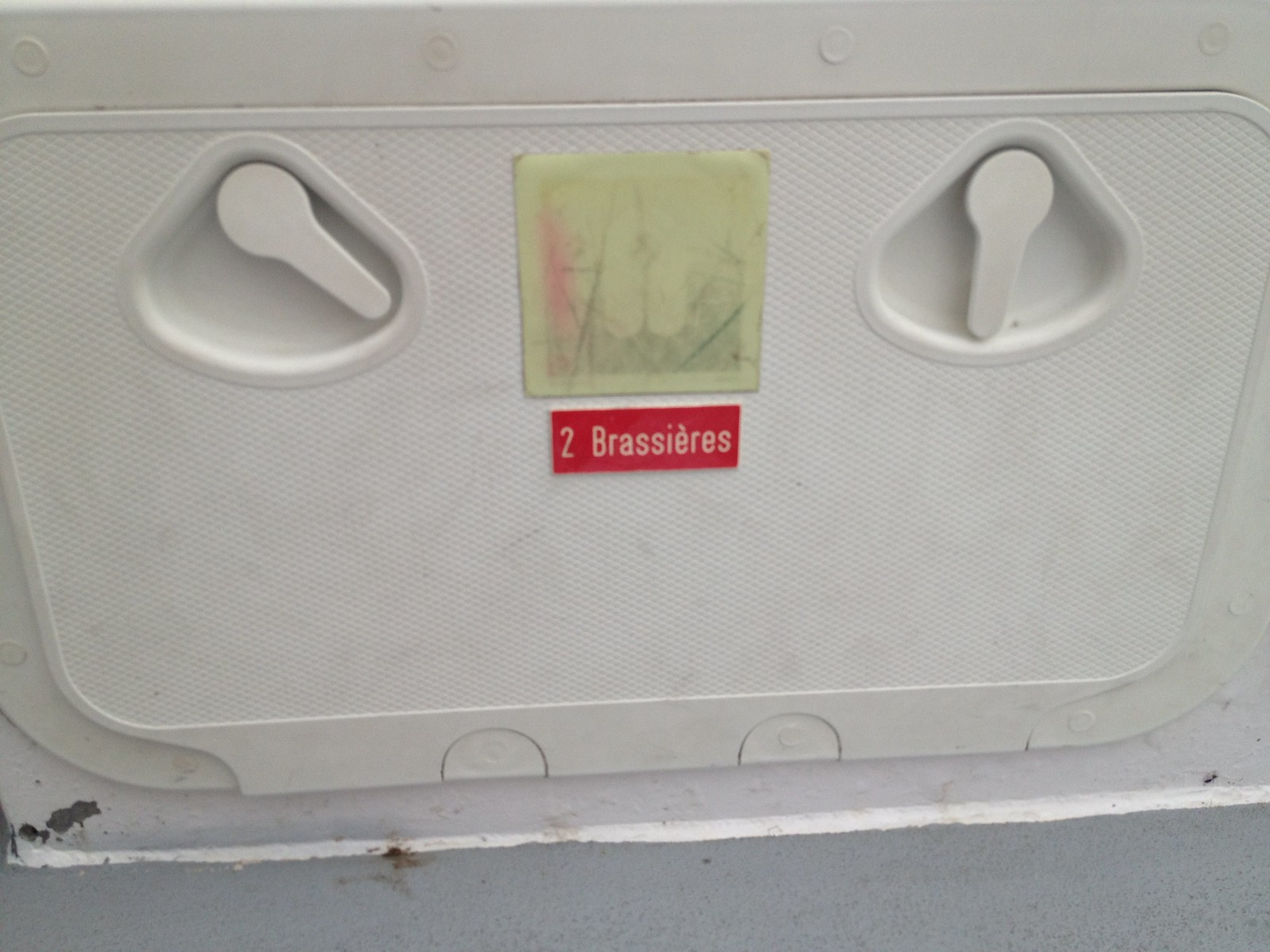The image features a close-up of a white storage compartment door, surrounded by a slightly dirty off-white wall with a gray strip at the bottom. The door, which shows signs of wear, has two quarter-circle recessed areas at the top, each holding a flat, spoon-shaped latch. The left latch is turned to the right, while the right latch is positioned vertically, pointing downward. Between these latches, there is a faded and scratched label plate that appears to depict a personal flotation device. Below this plate, a red plaque with white engraved text reads "Two Brassieres." The bottom left corner of the wall shows peeling paint, revealing the gray surface beneath.